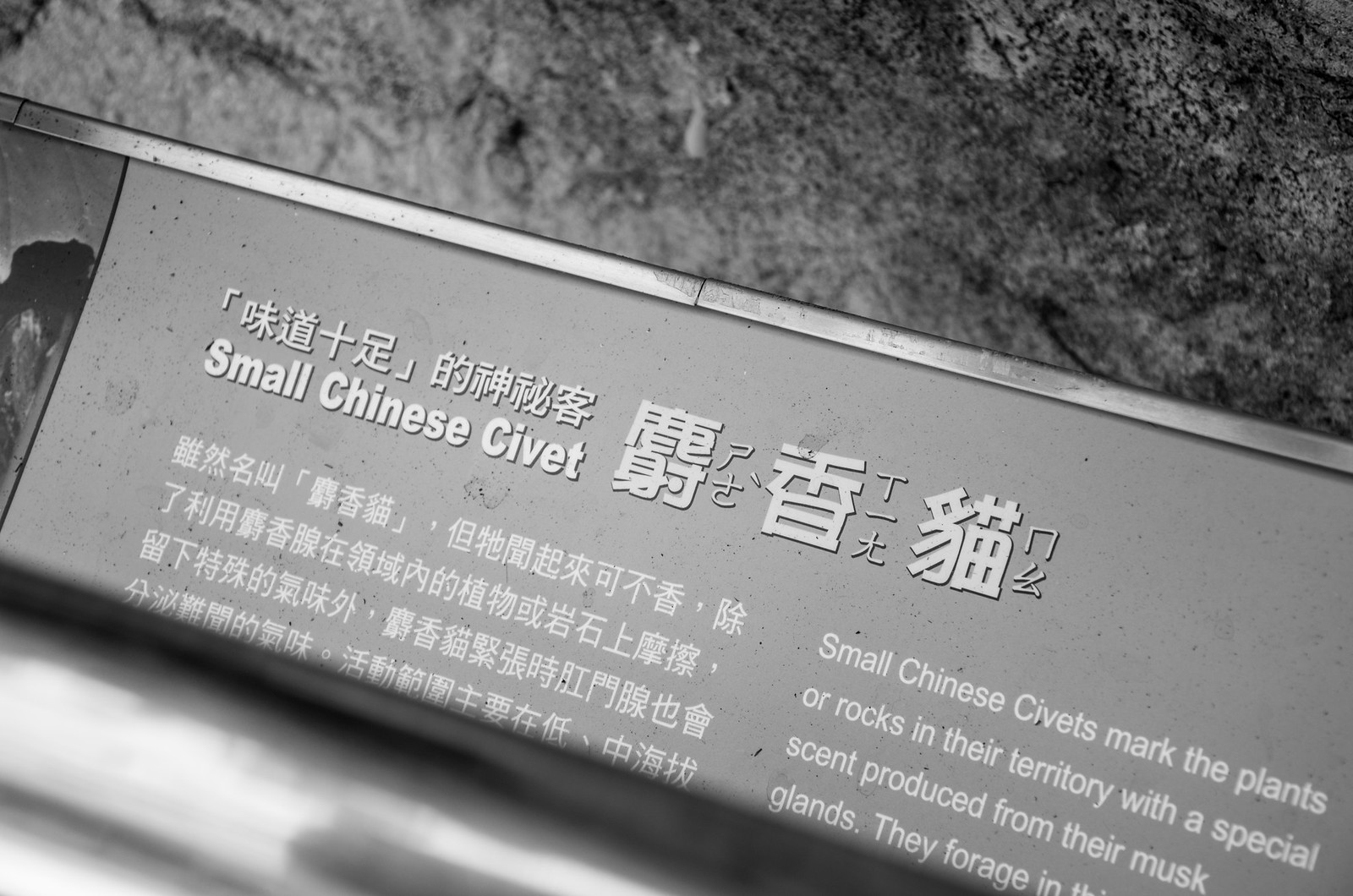This black-and-white photo appears to capture a sign or display likely positioned in a zoo or similar establishment, detailing information about the small Chinese civet. The top half of the image features a rocky backdrop, suggesting it is taken outdoors near a habitat, potentially a cave environment. The sign itself is rectangular and includes both Chinese and English text. The prominent English heading reads "Small Chinese Civet," followed by a paragraph stating, "Small Chinese civets mark the plants or rocks in their territory with a special scent produced from their musk glands." Unfortunately, the text cuts off after "they forage in the..." making the rest of the details unreadable. The sign is also accompanied by Chinese characters, with additional translations positioned to the right. The overall appearance includes white, black, gray, and silver colors, presenting a somewhat faded and grainy texture. The intricate mix of languages and symbols suggests an informative piece intended to educate visitors about the civet’s behavior and habitat.